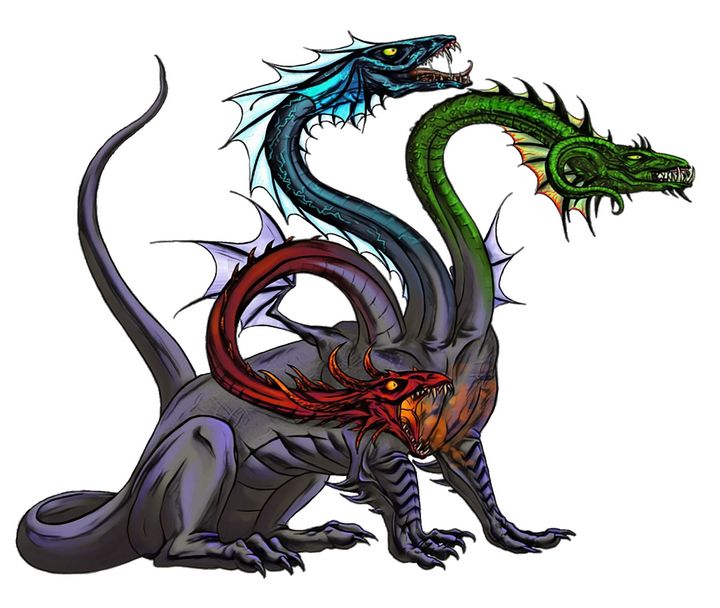The image is an illustration of a three-headed dragon, or hydra, set against a plain white background. The dragon's body is a blend of grayish-purple hues with black stripes on its four legs, each ending in long, sharp purple claws. The creature is depicted sitting on its rear, exuding an imposing presence with its distinctive, multi-colored heads.

The head on the left is red, adorned with sharp, upward-tilted horns. It is captured mid-roar, a red-orange glow emanating from its open mouth suggesting it is about to breathe fire. This head's neck is predominantly red.

The central head is blue, resembling a sea serpent with light blue fins along its neck and back. This head is the tallest and also has its mouth open, revealing rows of sharp white teeth set in a powerful jaw, and it sports piercing yellow eyes.

The head on the right is green and features curled, goat-like horns of the same color. Unlike its counterparts, this head has its mouth closed, though its sharp teeth are still visible. The eyes are squinted and yellow, and green tentacles extend from where its ears would be, adding a mythical quality.

The entire creature is detailed meticulously, from the texture of its scales to the menacing glare of its three pairs of yellow eyes, making it a formidable and striking figure.